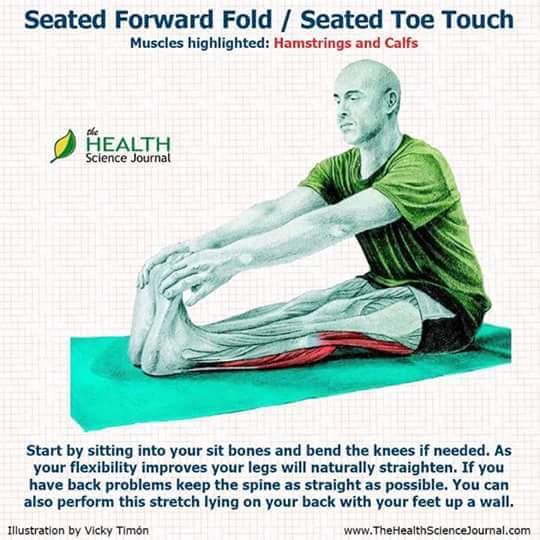The image is a detailed illustration from the Health Science Journal, showcasing a man performing the Seated Forward Fold, also known as the Seated Toe Touch stretch. The exercise is designed to target the hamstrings and calves, which are highlighted in red within the image. The bald man is depicted in a semi-robotic style, allowing a clear view of the engaged muscles. He is sitting on a green mat, wearing a matching green shirt. The instructions accompanying the image advise starting the stretch while sitting into the sit bones and bending the knees if necessary. It explains that as flexibility improves, the legs will naturally straighten and suggests keeping the spine straight for individuals with back issues. Additionally, it mentions an alternative method of performing the stretch by lying on the back with feet up against a wall. The illustration, credited to Vicki Timone, includes a logo of the Health Science Journal and features the text, "Seated Forward Fold/Seated Toe Touch," with the website www.thehealthsciencejournal.com indicated at the bottom for further reference.